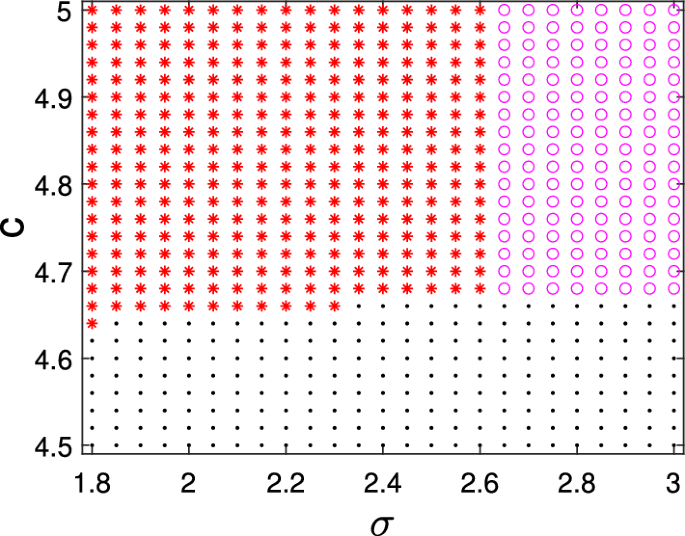The image is a detailed computer-generated rectangular graph outlined in black. The y-axis is labeled with a 'C' and ranges from 4.5 at the bottom to 5 at the top, marked in increments of 0.1. The x-axis, labeled with a Greek letter resembling a slanted zero with a line from the top, ranges from 1.8 to 3 in increments of 0.2. The graph itself features three distinct data regions: black dots span from the bottom left to just past the center, transitioning to tiny red starbursts, and finally, the upper right region is filled with purple circles that have white centers. This color-coded point arrangement indicates varying results across the two variables plotted on the graph.